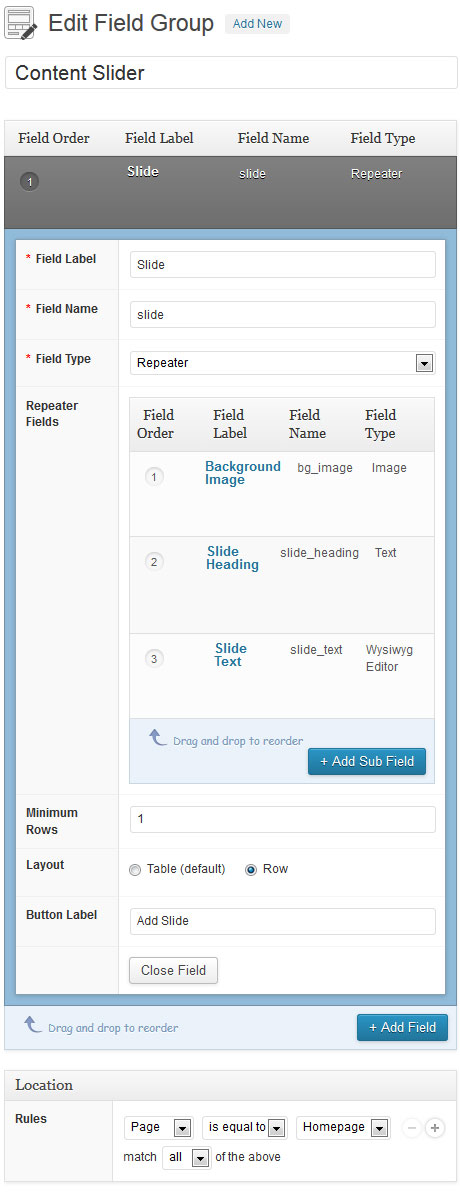The screenshot appears to be from a utility page used for configuration, possibly related to software or website settings. The overall background of the page is white.

### Top Section:
- **Top Left Corner:**
  - **Text:** "Edit Field Group" in dark gray font.
  - **Icon:** A small square with a pencil next to it, indicating an edit function.
  - **Button:** To the right of "Edit Field Group," there's a tiny gray rectangle with "Add New" written in blue letters.

### Content Area:
- **Primary Heading:** "Content Slider" located beneath the edit icon and button area.
- **Menu Bar:** Below this heading, a light gray menu specifies:
  - **Labels:** Field Order, Field Label, Field Name, and Field Type.

### Configuration Panel:
- **Menu:** There is a medium to dark gray horizontal menu with three items. The first item is labeled "Slide" in white text, the second item is illegible, and the third item starts with an "R" but is also unreadable.
  
- **Editable Area:**
  - **Outline:** Enclosed within a blue-outlined vertical rectangle, signifying the active configuration area.
  - **Sidebar Labels:** On the left sidebar:
    - Field Label
    - Field Name
    - Field Type
    - Repeater Fields
    - Minimum Rows
    - Layout
    - Button Label

- **Main Content:**
  - **Middle Menu:** A menu in a very light gray background with headers: Field Order, Field Label, Field Name, and Field Type.
  - **Entries:** Beneath this menu, there are three items listed, which seem to be names of image files.

### Bottom Section:
- **Rules:** At the very bottom left, there is a label "Rules."
  - **Dropdown Menu:** Next to "Rules," a dropdown menu labeled "Page" with an arrow indicating options. The configuration specifies "is equal to Home Page" with an additional condition of "Match All."

This detailed caption provides a thorough description of the utility page screenshot, capturing all visible elements and their arrangement.